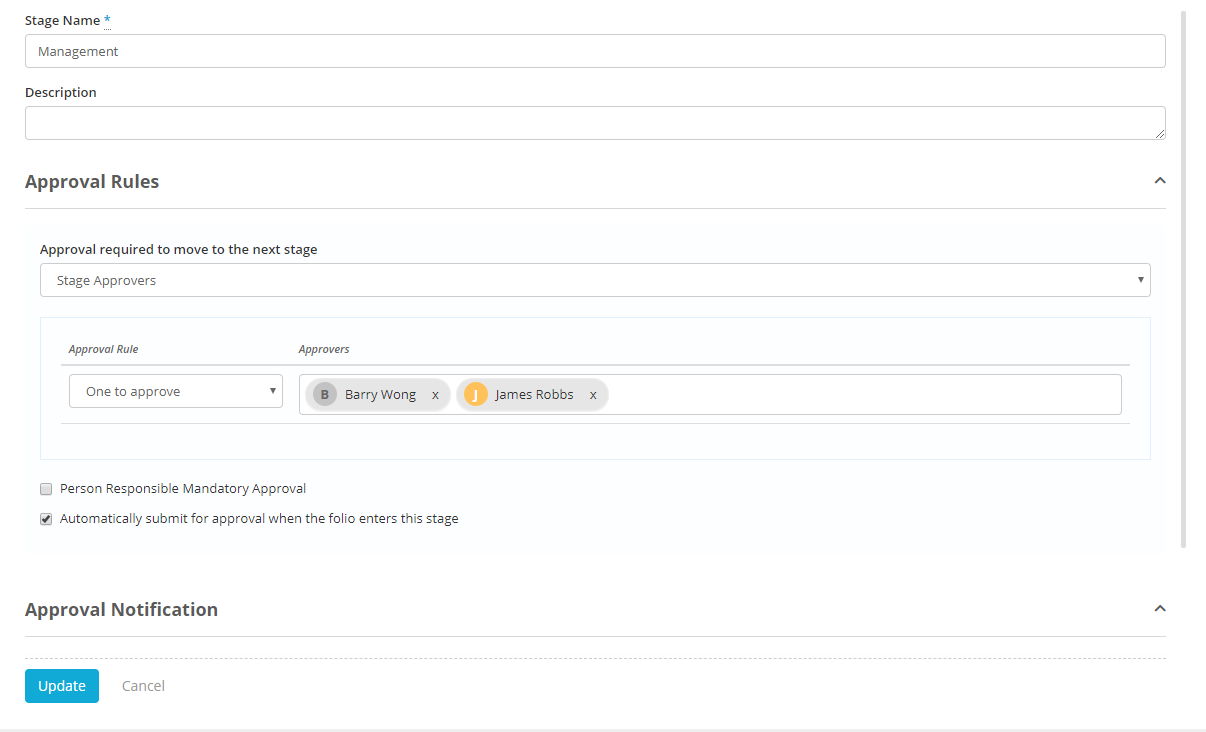The image displays a detailed project management interface highlighting the approval process for different stages. At the top, within a blue star, is the "Stage Name" field, labeled "Management." Below, there's a section for the "Description," followed by a list of "Approval Rules."

A rule specifies when approval is required to move to the next stage, and the interface includes a dropdown menu for selecting stage approvers. This section resembles a table and contains columns labeled "Approval Rule," "Approvers," and "When to Approve." In one of the dropdowns, the name "Barry Wall" is highlighted with a yellow circle, while "James Robbs" is marked within an oval shape.

Further down, there's an option for marking a person as responsible for mandatory approval. There’s also a checkbox for automatically submitting for approval once the image reaches the full stage. Notifications are handled via a rectangular button labeled "Update," and there's an "Cancel" button at the bottom in green. The top of the interface is marked with dashed lines, completing the structured outline of the approval system interface.